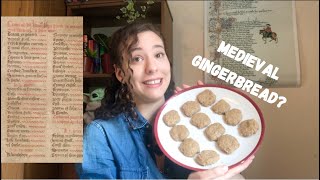In this image, a woman with long, partially curly hair cascading over one eye stands in her kitchen, holding up a large white plate with a red rim, adorned with a dozen brown, round cookies. The arrangement of cookies, possibly medieval gingerbread, is accentuated by the visible text "Medieval Gingerbread?" in block letters on the plate. She wears a denim shirt with a collar and has a pensive expression, her smile appearing somewhat forced or worried.

Behind her, the kitchen walls are tan-colored, and a round shelf unit displaying various items, including a toy Yoda peeking out near her shoulder, adds context to the setting. Additionally, there’s a picture on the wall featuring a horse and extensive writing. To the left of her, there appears to be a blurry, ancient recipe, which might be related to the cookies she is presenting. The environment and details suggest she's sharing or contemplating an old recipe within the comfort of her home.